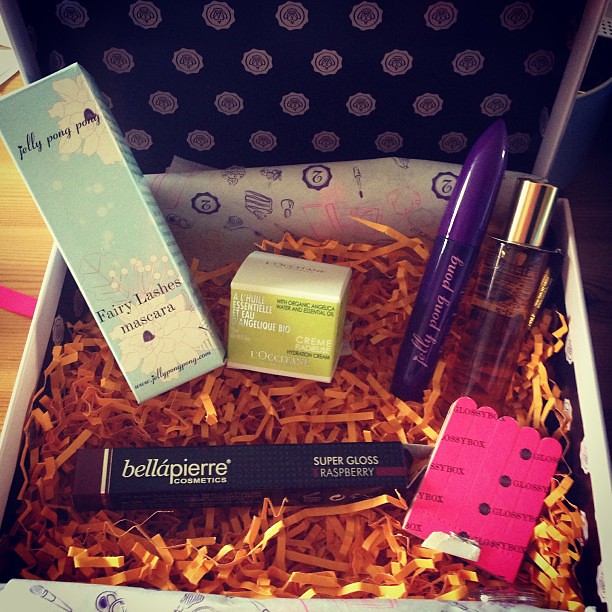In this close-up photograph taken from above, you see a gift box filled with various beauty products, all nestled on a bed of shredded orange crinkly paper. Dominating the left side of the box is a light blue and white rectangular product box labeled "Jelly Pong Pong," featuring "Fairy Lashes Mascara" in black text. Below this, towards the bottom of the box, there's another rectangular blue box with a purple end, which reads "Bella Pierre Cosmetics" and "Super Glossy Raspberry." To the right, a small squat green and white box is visible, somewhat blurred but seemingly labeled "Essential Bio Cream." Just beside it lies a metallic or purple tube. At the far right of the box is a clear container with a gold lid, possibly containing a fragrance. On the bottom right, a cluster of hot pink emery boards marked "Glossy Box Alarm" is seen. The inside lid of the box is dark blue, decorated with purple crown images, and part of a light brown, wood-grain table is visible in the background.